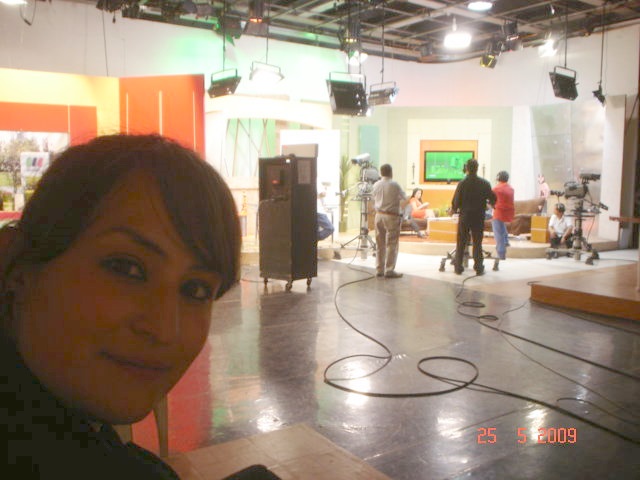The photograph captures an indoor television studio set with an array of lighting equipment suspended from the ceiling, all aimed towards a corner of the room that occupies the upper-right portion of the image. In the lower-left corner and close to the camera, a woman with brown hair parted to the side, dark eyes, and wearing a dark top smiles directly at the viewer. She appears to dominate the foreground, potentially as the one taking the picture or being prominently featured. Towards the middle-right section of the image, a woman with dark hair is seated on an orange couch, preparing to record a segment. Surrounding her are several individuals, presumably crew members, positioned near camera and other filming equipment. Additionally, a monitor displaying a green screen is visible on the wall behind the setup. The studio floor is crisscrossed with various cables connecting the equipment, contributing to the bustling atmosphere of the set. Notably, in the lower-right corner of the photograph, there is a timestamp reading "25-5-2009."